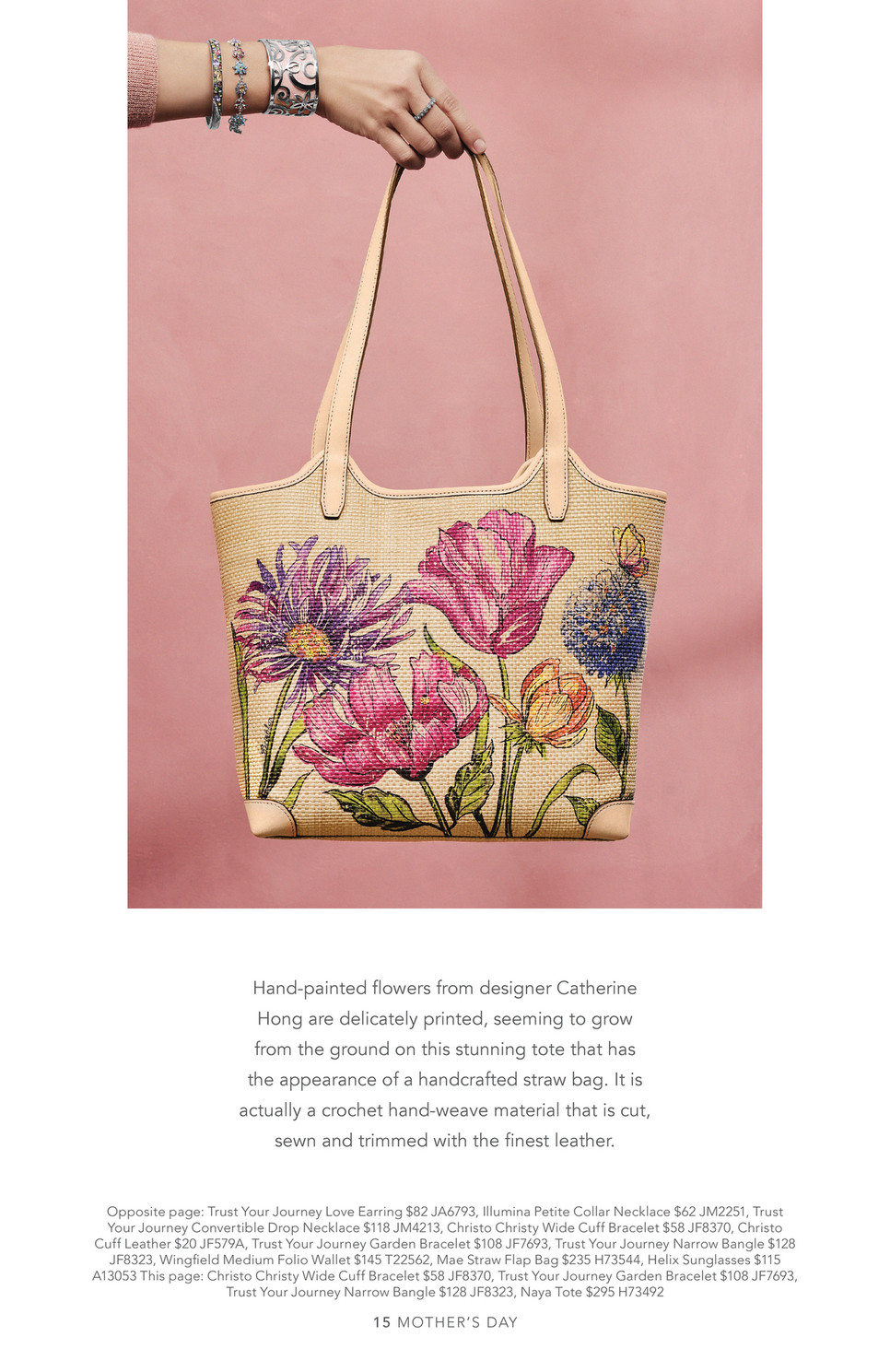The image displays a beautifully designed tote bag with a handcrafted feel. The bag, reminiscent of a tan-colored handcrafted straw bag, is actually made from intricately crochet hand-weave material, skillfully cut, sewn, and trimmed with the finest leather. It features exquisite hand-painted flowers in shades of pink, purple, yellow, and blue, delicately printed by designer Catherine Hung. The floral designs appear to grow naturally from the base of the tote, enhancing its artisanal appeal. This picture showcases a woman's hand, adorned with various bracelets and a ring, emerging from the top left corner, holding the tote by its long strap. The backdrop is all pink, and the person is wearing a pink sweater, complementing the purse and its details. Beneath the image, there is a substantial amount of text; the top part describes the designer and the tote's features, while smaller text below likely provides additional information about the product and its price.